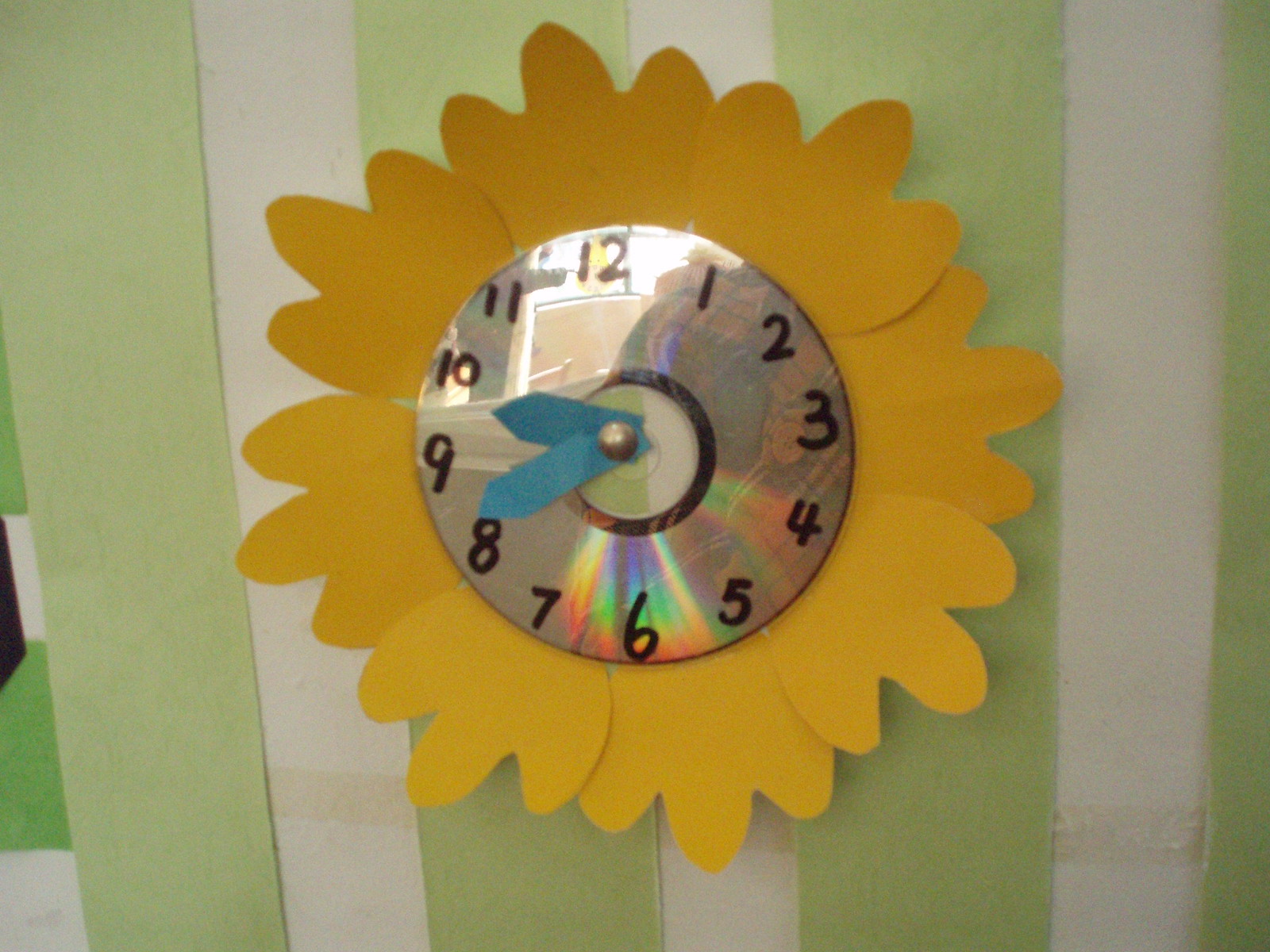The picture features a creatively crafted clock made primarily from construction paper and a CD. The clock face, situated in the center of the image, is a repurposed CD reflecting part of a shirt and chair. Around the CD, the numbers 1 through 12 are meticulously drawn, resembling a traditional clock. The clock hands are fashioned from blue construction paper and secured at the center by a silver thumbtack. The shorter and longer hands indicate the hour and minute, respectively.

Encircling the CD are eight yellow construction paper petals, arranged to give the appearance of a sunflower, with two shorter petals on the outside bracketing one slightly longer petal in the center, repeating this pattern all the way around.

The clock is mounted against a green and white striped wall, made from alternating vertical strips of construction paper—four green stripes and three white stripes. To the left of the clock, additional fragments of construction paper—white, green, and a hint of black—peek into the frame, extending to the edge of the image.